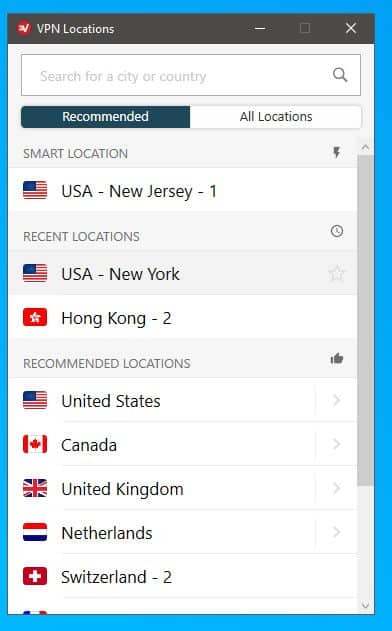Detailed Descriptive Caption:

The image depicts a mobile application interface for selecting VPN (Virtual Private Network) locations. At the top of the screen, the heading "VPN Location" is prominently displayed, indicating the app's function of allowing users to choose their desired virtual location. The main screen is segmented into three subsections: 'Smart Location,' 'Recent Locations,' and 'Recommended Locations.' 

Under 'Smart Location,' the app suggests "USA, New Jersey," likely due to its proximity to the user's physical location, providing the fastest connection. The 'Recent Locations' section lists "USA, New York" and "Hong Kong," places the user recently connected to. The 'Recommended Locations' section offers a variety of options including the US, Canada, UK, Netherlands, and Switzerland, with more locations accessible by scrolling down.

The user interface has a clean design with a predominantly white background and subtle light gray elements for visual contrast. A blue border frames the app window, giving it a polished look. The image appears to be cropped, focusing on the central features of the VPN location selection screen.